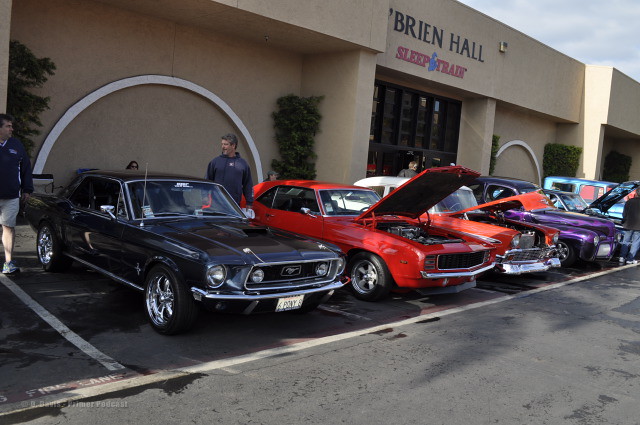The photograph captures a lively car show set in a parking lot in front of a large, light brown, whitish building that prominently reads "O'Brien Hall" in black letters, with "Sleep Train" in red letters below. The building features black double doors and is adorned with manicured bushes and tall trees. A row of colorful classic cars, invoking a sense of the 1960s sports car design, is parked in marked spaces on the black pavement. These include a black classic car, a custom red car resembling an old Chevy Malibu with a white roof, a bright orange car, and a metallic purple car. The hoods of the cars are mostly open, allowing for close inspection, except for the black and purple vehicles. A man in a black, long-sleeve, button-up shirt stands near the black car, seemingly conversing with another individual walking away to the left side of the frame. The scene is a vibrant showcase of automotive history against the backdrop of the "O'Brien Hall Sleep Train" building.